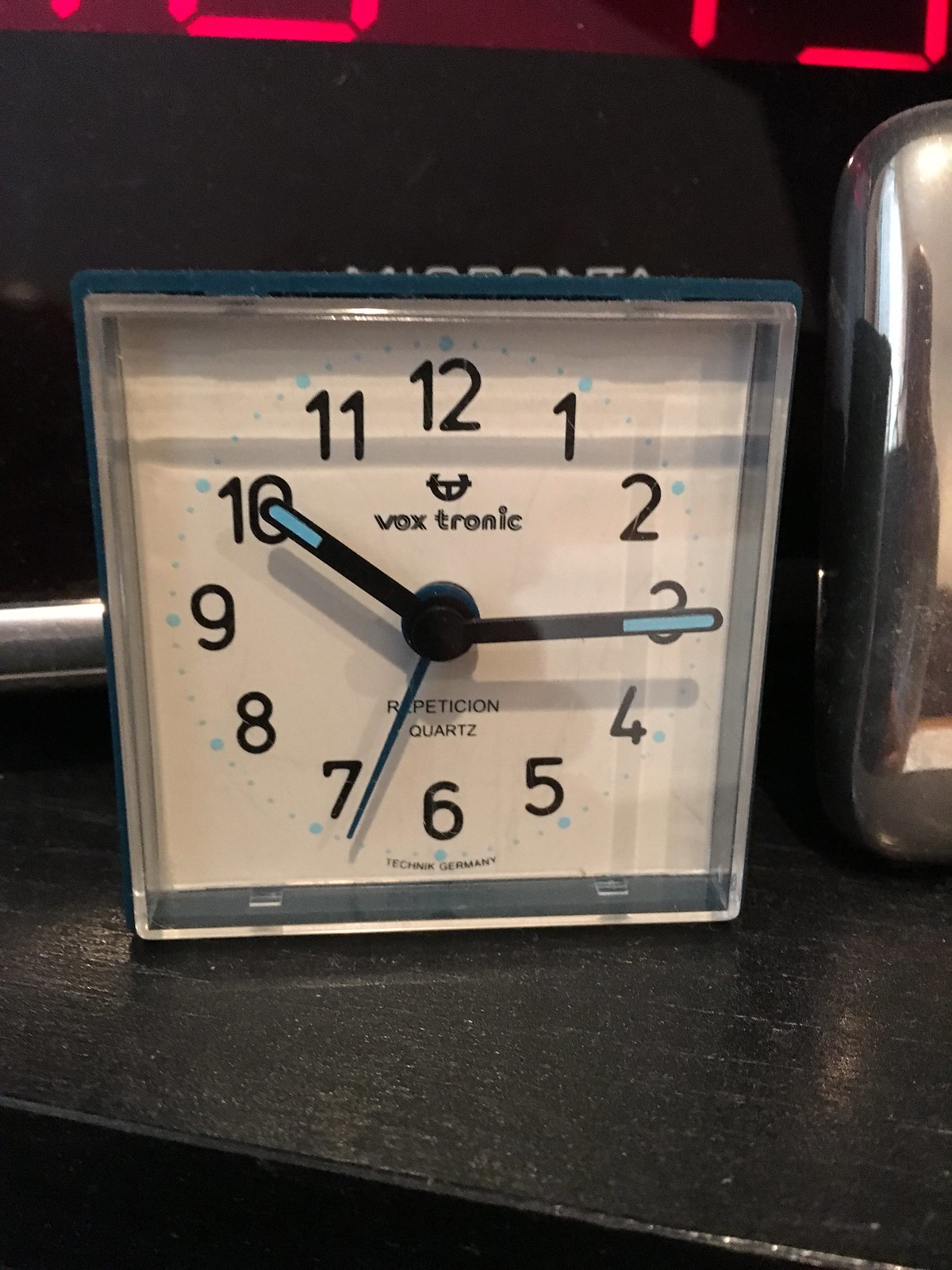In this image, we see a clock prominently displayed on what appears to be a dark wood or possibly black tile shelf. The clock is square-shaped with a silver frame and a face protected by a glass or clear plastic panel. The face of the clock is white, with black numbers from 1 to 12 arranged in a clockwise direction. There are small teal blue dots marking the increments between the numbers. The hour and minute hands are black with blue tips, while the second hand is solid blue and currently pointing near the 7, indicating the time is approximately 10:15:35. Above the center of the clock face, the brand name "Voxtronic" is visible, along with the word "Quartz" beneath it. In the very top sliver of the image, there is a hint of red digital numbers, which are not fully visible, adding an element of intrigue. To the right of the clock, there appears to be a silver object whose identity remains unknown.